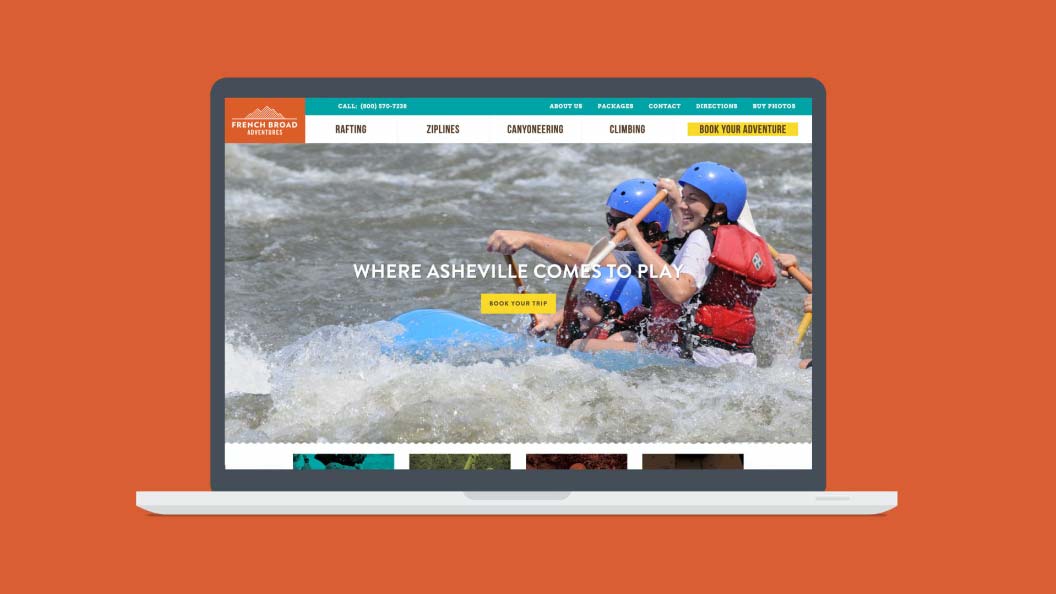The image features an artistic drawing set on a burnt orange background that depicts a laptop with its screen open, displaying a website. The laptop drawing includes a white bar at the bottom, signifying the edge of the keyboard, and the screen is outlined in dark grey.

On the laptop screen, there is a rendered website interface. In the top left corner of the site, there is an orange logo adorned with some text and an indistinguishable element above it. Spanning the top of the screen is a dark turquoise bar on which a number and five menu options are visible, starting from the center and extending towards the top right corner.

Beneath this, a white navigation bar is present that houses five options: the first resembling a rafting icon, the second resembling a zip line, the third is unclear, the fourth is related to climbing, and the fifth is not legible. On the far right of this navigation bar is a prominent yellow button labeled "Book Your Adventure."

The principal part of the website displays an engaging photograph of individuals kayaking in a whitewater rafting scenario. Superimposed on this image, in the center of the screen, is the slogan "Where Asheville Comes To Play," accompanied by a smaller yellow button below it that reads "Book Your Trip." At the bottom of the screen, four thumbnail images are visible, though their details are too small to discern.